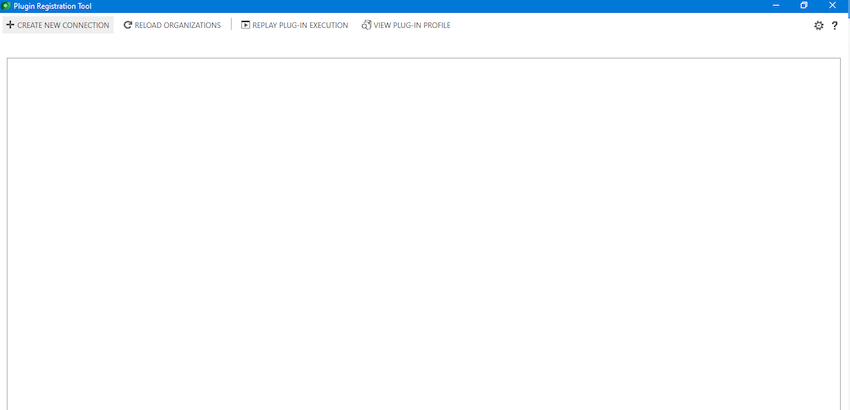In this image, the top section features a horizontal blue line. At the left end of this line, there is text in white font that reads "Plug-in Restoration Tool," accompanied by a small green square or dot, although it is barely noticeable due to its size. On the far right of the line, there is a short white vertical line followed by a white box and a white "X."

Beneath this, on the next line down, there is a gray box on the left with gray font that includes a "+" symbol and the words "Create New Connection." Adjacent to this, there is an icon of a reload button accompanied by the text "Reload Organizations." 

To the right of these elements, there is a box containing a black triangle pointing to the right, labeled "Replay Plug-in Execution." Further right, on the same line, there is text that reads "View Plug-in People," although the accompanying image is unclear.

On the extreme right, there are icons for settings and a question mark. Below this entire section is an incomplete gray square with its bottom side missing, set against a white background.